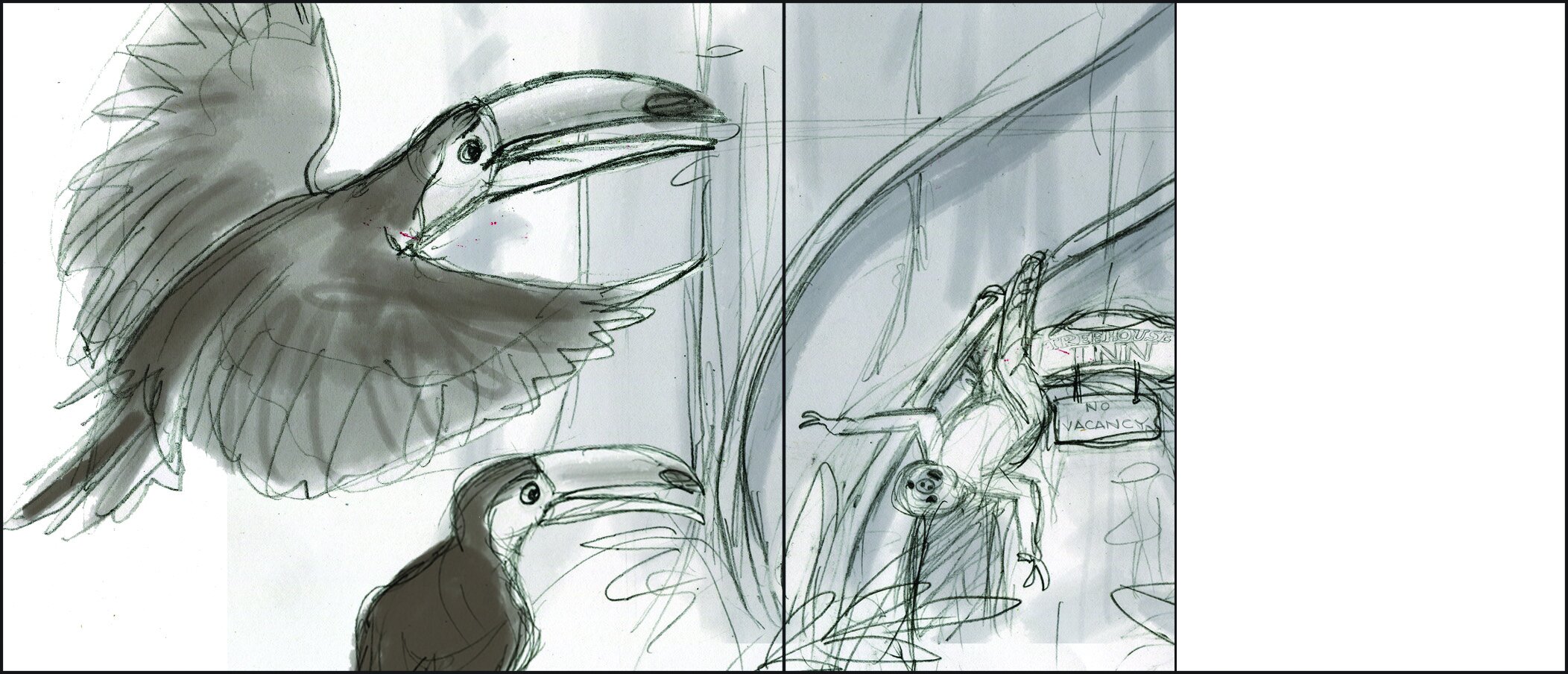This is a detailed black-and-white hand-drawn illustration depicting two toucans. One toucan is mid-flight with its wings spread wide, while the other toucan appears to be perched, though not clearly on what, as the picture is cut off. Both birds have large, distinctive beaks and attentive eyes, seemingly staring through a window. On the other side of the window, there is an upside-down human figure, drawn with scribbled, quick lines, suggesting a fast and expressive rendering. The person appears to be falling or perhaps suspended in an unnatural pose, adding an element of surrealism to the scene. Behind this figure, a sign reads "No Vacancy" with an accompanying partial sign indicating a hotel or motel setting. The composition uses various shades of black, gray, and white to create depth and texture, making it an intriguing and somewhat eerie piece.